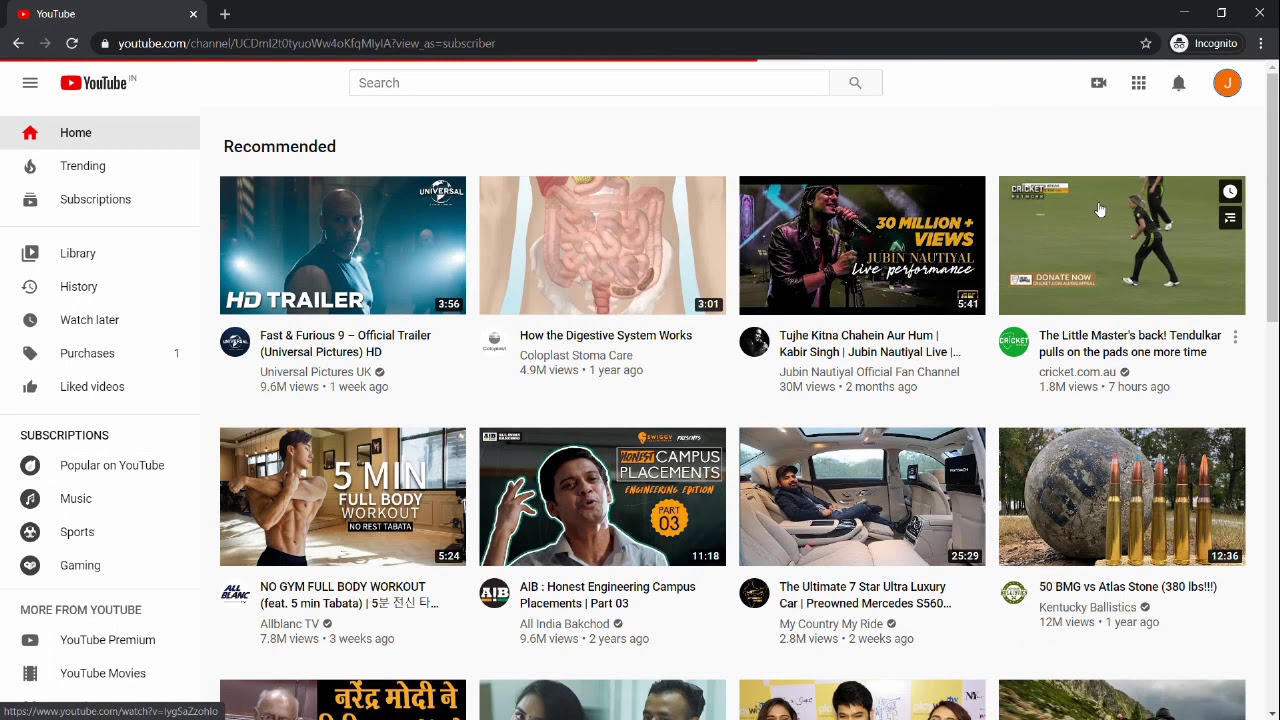This detailed horizontal screenshot captures the YouTube website in a web browser interface. A dark gray header bar spans the top of the screen, featuring multiple navigation elements, including a left arrow, a refresh button on the left, and an incognito mode button on the right. An address bar is positioned centrally within the header.

Directly below this header, the YouTube page layout begins with the iconic YouTube logo, a prominent search bar, three icons, and a user profile represented by the letter 'J' within an orange circle. A vertical scroll bar on the right side indicates additional content below the current view.

On the left-hand side of the screen, a navigational sidebar includes various sections labeled with both text and icons. These sections are organized from top to bottom starting with: Home, Trending, Subscriptions, Library, History, Watch Later, Purchases, and Liked Videos. Further categories listed include Popular on YouTube (featuring Music, Sports, Gaming), and More from YouTube (featuring YouTube Premium and YouTube Movies).

The main content area showcases a grid of twelve video thumbnails, though only eight are fully visible at the top section of the screenshot. The identified video titles in the top row are: "Fast and Furious 9 Official Trailer," "How the Digestive System Works," "To He, Kitna, Chahine," "Our Home," and "The Little Master's Back." These video recommendations suggest a diverse range of content tailored to the user’s interests and YouTube’s algorithm.